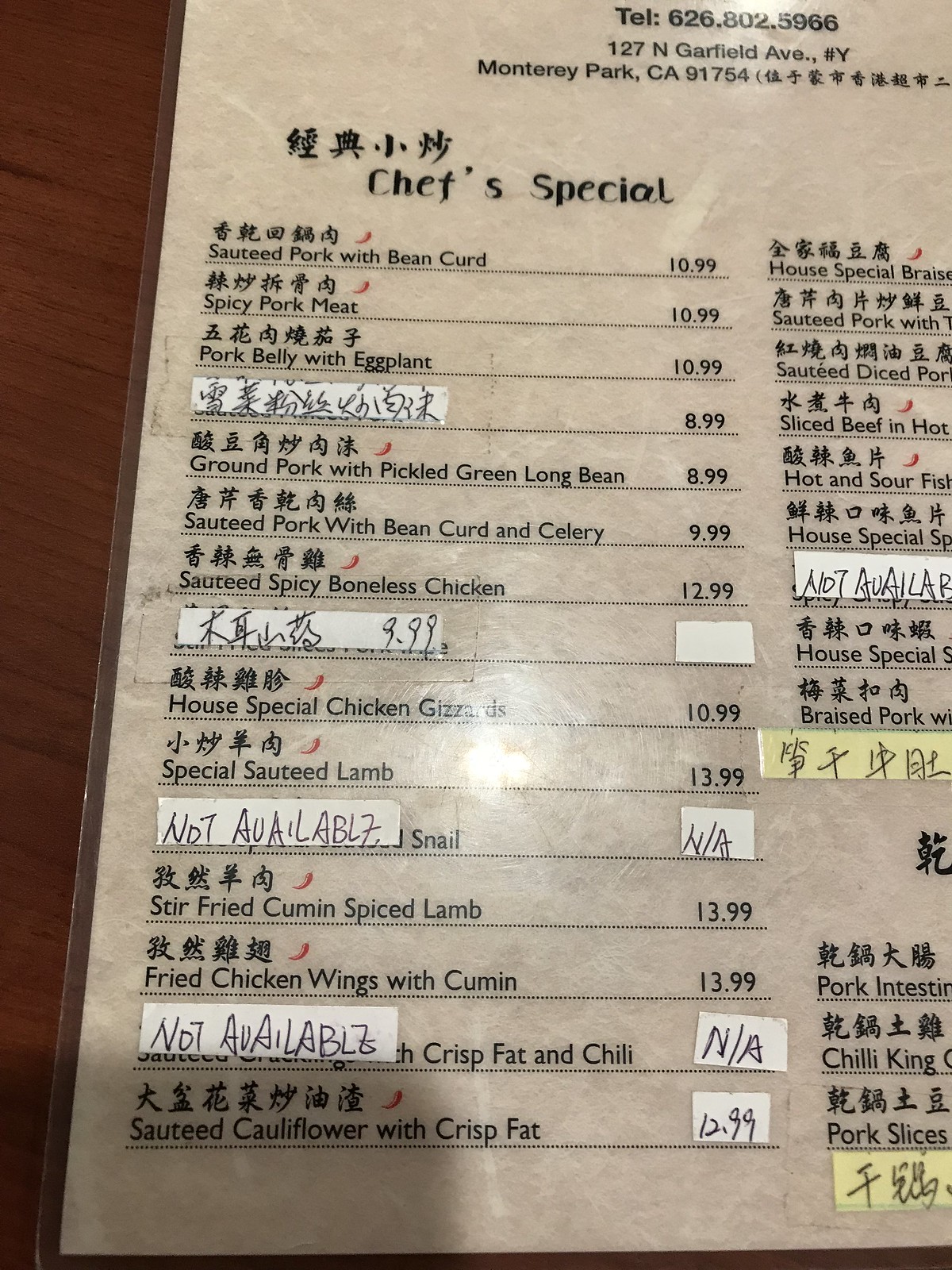This image is a color photograph taken from above, depicting a laminated menu from an Asian, likely Chinese, restaurant. The light source from above creates a reflection at the center, slightly below the middle of the image. The menu occupies two-thirds to three-quarters of the left vertical side of the frame, with the remaining portion cut off by the right edge. 

At the top of one visible column, the heading "Chef's Special" can be seen, underneath which an array of dishes is listed. Notable items include sautéed pork with bean curd, sautéed spicy boneless chicken, stir-fried cumin spiced lamb, and sautéed cauliflower with crisp fat. 

Numerous white labels with handwritten text in black ink cover portions of the menu, obscuring some dish names and prices. Some of these labels are inscribed in an Asian language. Notably, a few labels at the bottom read "not available." The right side of the menu also features additional white stickers indicating items that are unavailable, along with two yellow stickers.

The menu includes the restaurant's contact information, situating it in Monterey Park, California.